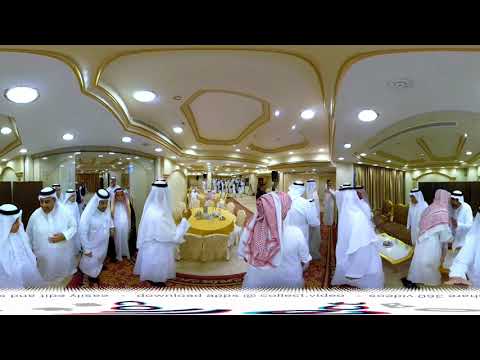This panoramic image captures an event within an ornately decorated hall, likely a hotel conference center, filled with Middle Eastern men in traditional white robes and white head coverings secured with black bands. The interior features a white ceiling with gold trim and elaborate detailing, adding a sense of grandeur. The men are congregating, talking, and gesturing to one another, with some wearing red scarves over their head coverings. They are spread throughout the space, which is divided into three sections. Dominating the middle section is a yellow circular table adorned with an ornate centerpiece and surrounded by yellow fabric chairs. Additional elements include a gold curtain in the background and a hallway seen on the far left. The atmosphere suggests a formal ceremony or gathering, with intricate decorations and an air of anticipation as no one has yet taken their seats.